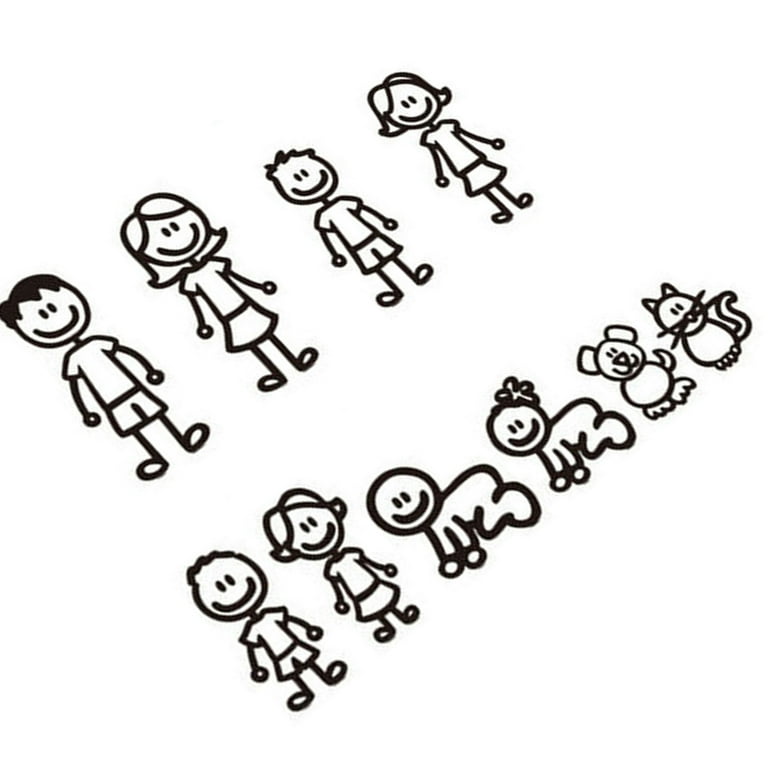This image showcases a playful illustration reminiscent of the popular family stickers often seen on the back of minivans or cars. Arranged in two rows at a slight slant, the top row features a dad, a mom, and two school-aged children—a boy and a girl—all drawn in a simple, black marker style. The bottom row includes a toddler boy, a toddler girl, a baby boy, and a baby girl, alongside the family pets: a dog and a cat. The illustrations boast basic stick figure-like bodies with smiling faces, capturing a cheerful and whimsical family vibe, though the cat intriguingly lacks a smile. This composition likely hints at a customizable sticker set designed for vehicle adornment, offering a way to proudly display the makeup of one's family.